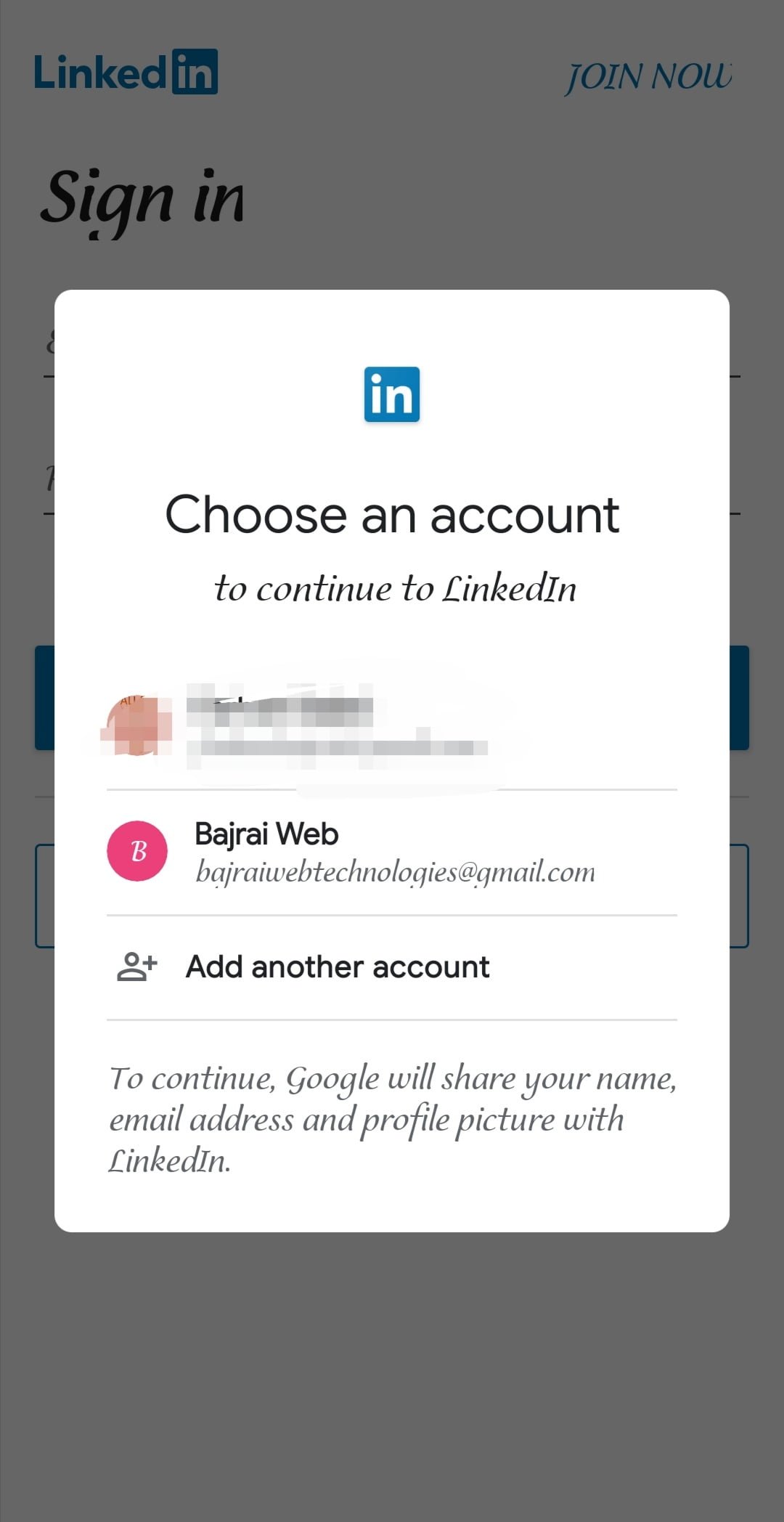This detailed descriptive caption conveys all the visual elements and textual content observed in the image:

---

Screenshot of a LinkedIn login page. The background is gray. At the top left corner, the LinkedIn logo is displayed, with "Linked" in blue and "IN" in white inside a blue square. To the right, there is a "JOIN NOW" button in blue, written in all caps. 

About three lines below the LinkedIn logo, the "Sign in" text is bolded in black. Below it, a white rectangular input area is visible, and at the top center, a blue square outlined in white with a lowercase white "IN" is displayed.

Two lines below that, centered in black, the text "Choose an account" is written. In a different, slightly slanted font, the phrase "to continue to LinkedIn" appears in gray two lines under the previous text.

Below this, a profile circle on the left, which appears orange, has its associated black writing blurred out. Underneath this, another hot pink profile circle with a white capital "B" inside it is visible. To the right of this circle, the text "B-A-J-R-A-L Web" is bolded in black, and light gray writing appears below it.

Further below, on the left, there is a gray icon consisting of a person-shaped circle on top of a small flat rectangle with a plus sign. To the right of this icon, the text "Add another account" is bolded in black. Below this text, in gray, it says "To continue, Google will share your name, email address, and profile picture with LinkedIn."

---

This caption effectively describes all the elements present in the screenshot in a detailed and organized manner.